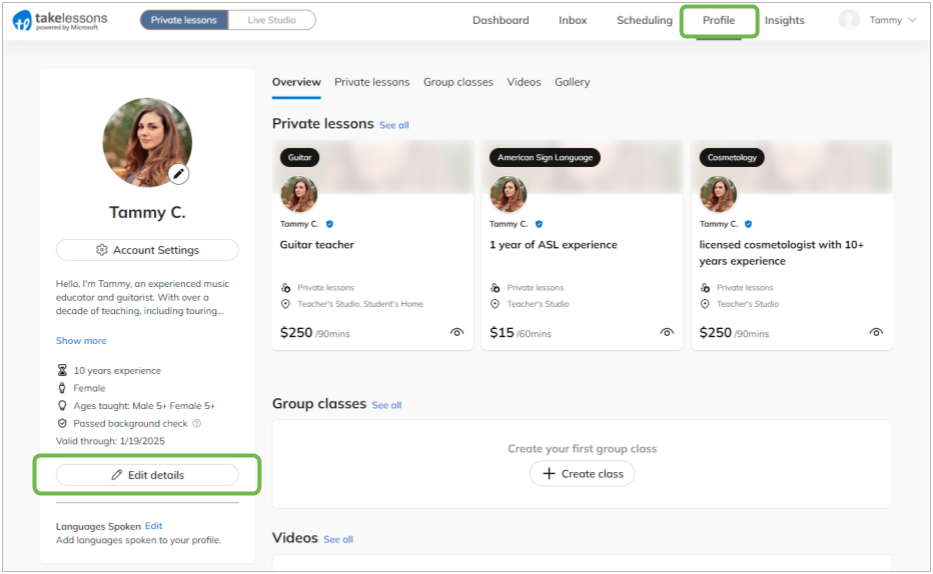In the screenshot of a webpage from the "Take Lessons" platform, we see various interface elements and user information. Located in the upper left-hand corner, there is a blue logo with the letters "TL." Next to it, the text "Private Lessons" is presented in white against a blue background. Below it, there are several tabs: "Dashboard," "Inbox," "Scheduling," "Profile," and "Insights," each on a white background with gray text. 

The user's name, "Tammy," is displayed prominently, and the "Profile" tab is highlighted in green. Within the profile settings, "Tammy C." is mentioned. Adjacent to this, there is a photograph of a woman with long brown hair. A brief introduction below the picture states, "Hello, I am Tammy, an experienced music educator and guitarist with over a decade of teaching, including touring," followed by a "Show More" hyperlink.

Additional details mention that Tammy has 10 years of teaching experience and can instruct both male and female students aged 5 and up. She has successfully passed a background check, valid through January 19, 2025. Lastly, there is a green "Edit Details" button indicating that Tammy charges $250 for a 90-minute guitar lesson.